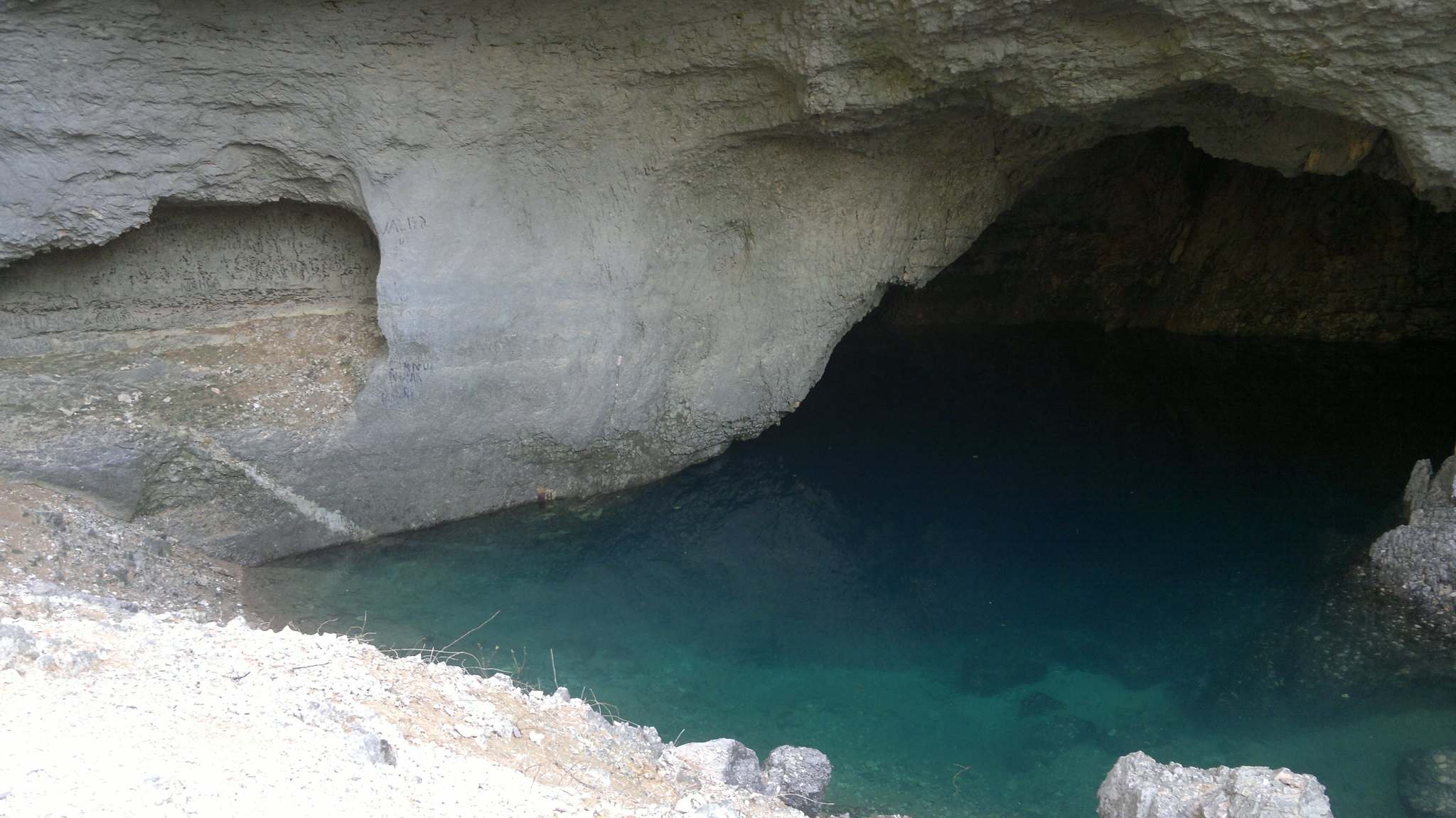The image depicts an intriguing underground grotto characterized by its dark, rocky cave formations made of gray, white, and brown stone. The water in the grotto glistens with a clear, bright blue-green hue, resembling a pristine oasis. The scene features a prominent, curved cave opening that allows sunlight to stream in, illuminating the entrance and making the water sparkle. However, as the cave extends deeper, the light diminishes, casting shadows and darkening the water to a deep, almost black color. The photo is devoid of any people or animals, focusing solely on the natural beauty and the serene, undisturbed atmosphere of the grotto and its crystal-clear waters.